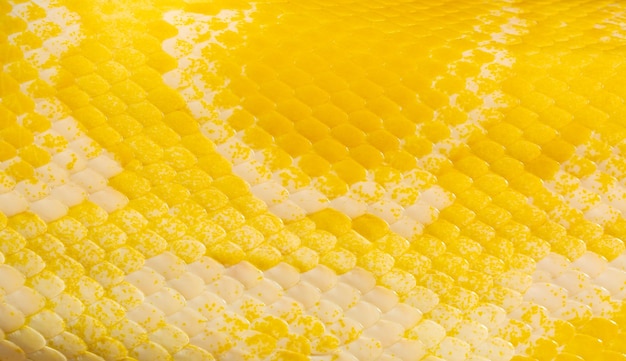This image is a close-up view of a snake's skin, predominantly featuring a vibrant, lemon-yellow color. The intricate scaly texture showcases tiny, tightly packed scales varying in shades of yellow and off-white. These scales create a striking, random pattern that can be likened to the appearance of corn kernels. White streaks and splashes intersperse the yellow, forming irregular lines and circles that traverse the image from the upper right to the center and around to the upper left, as well as vertically from the right center. The detailed arrangement of the scales and the interplay of colors highlight the unique and captivating design typical of snake skin.